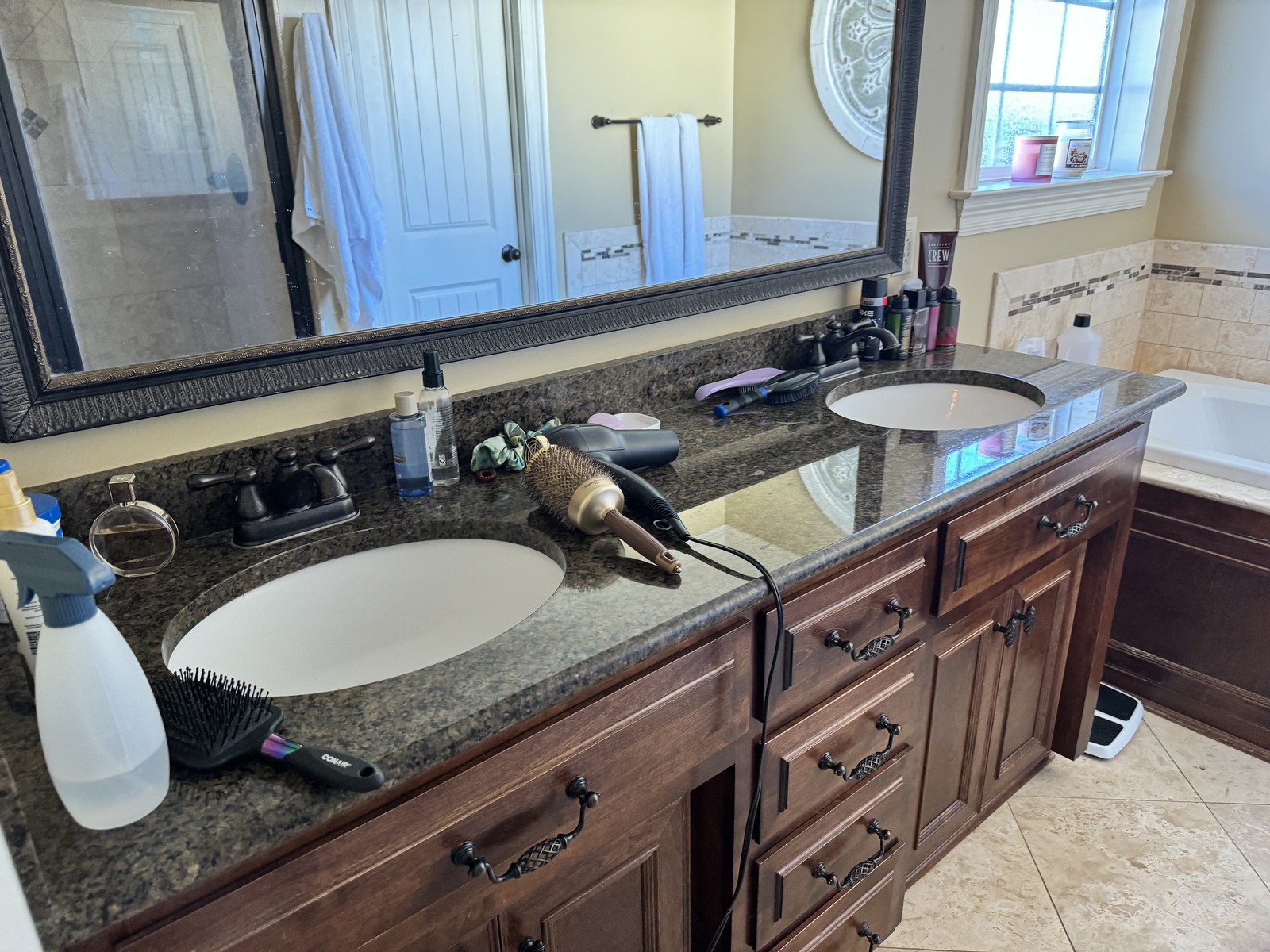The image depicts an elegant bathroom typically found in larger homes. Dominating the space is a substantial mirror affixed to the wall, reflecting the room's details. The double sinks feature a speckled, gleaming countertop, complemented by a dark brown cabinet base adorned with Victorian-style metal handles. Atop the counter, several personal care items are neatly arranged: a hairbrush, a spray bottle filled with liquid, a round container of fragrance, a small bottle with a blue label likely containing shampoo or soap, a large round hairbrush, and a sizable gray hair dryer. On the right-hand side, an assortment of bottles and two additional hairbrushes can be seen. The photo also partially reveals a bathtub on the right edge and a small portion of a scale on the floor. A window is visible in the upper right corner, lending natural light to the scene.